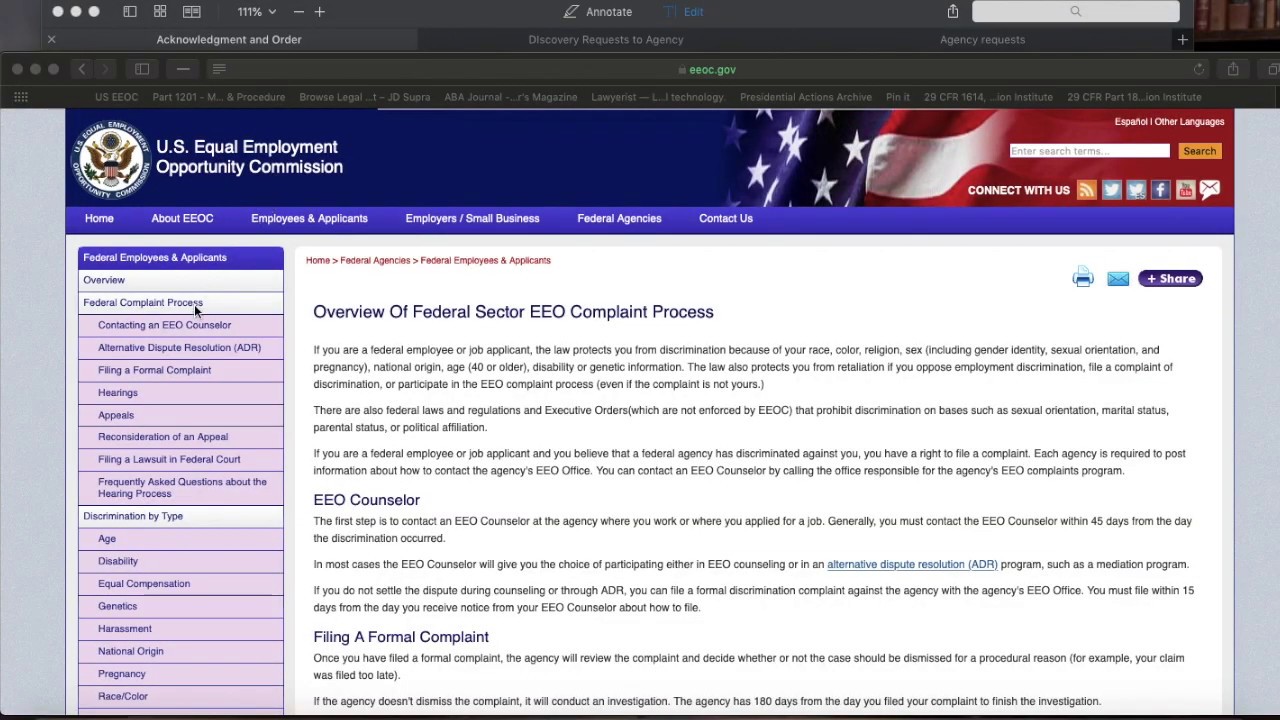The image is a screen capture of the U.S. Equal Employment Opportunity Commission (EEOC) website displayed on a device in landscape mode, possibly a computer or tablet, indicated by its width. The browser window features a dark gray bar at the top, housing tabs and navigation buttons. Below this, the website itself is presented with a clean, white background framed by gray strips on both the left and right sides.

Dominating the upper portion of the screen is a dark blue banner stretching across the top. On the left side of this banner, the text "U.S. Equal Employment Opportunity Commission" appears in bold white letters. Adjacent to this text is the official seal, showcasing a bald eagle clutching arrows and an olive branch, overlaid with a crest featuring the American flag. The right side of the banner prominently displays an image of the American flag, partially covered by a search bar and inclusive of social media icons.

Running vertically along the left edge of the screen is a lavender menu bar with black text, providing navigation options. The main content area of the website is primarily white with black text, interspersed with various colored links, including blue and red, for easy navigation. This structured layout ensures that the essential information and navigation tools are clear and accessible, reflecting the professional nature of the EEOC's online presence.